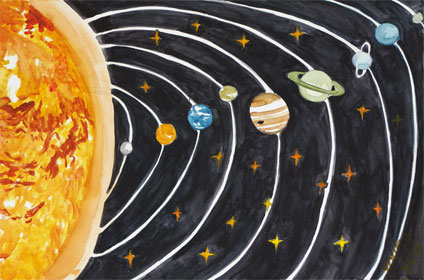This is a vibrant, cartoon-style drawing of our solar system on a black background. The black sky is dotted with numerous yellowish-orange stars, creating a sense of depth and wonder. A portion of the sun, radiating in hues of red and orange, appears on the left side of the image. Extending from the sun to the right are the planets, each distinct in color and size. The planets are aligned in the following order: the small, grayish Mercury; the slightly larger orange Venus; the blue Earth; the greenish Mars; the brown and white Neptune; the large green Jupiter with its iconic ring; the blue Saturn, which also features a ring; and finally, the distant blue-gray Pluto. White strips arc across the entire background, illustrating the orbital paths of the planets. The careful placement of stars, as well as the detailed depiction of planets and their orbits, makes this drawing a highly detailed and captivating representation of our solar system.